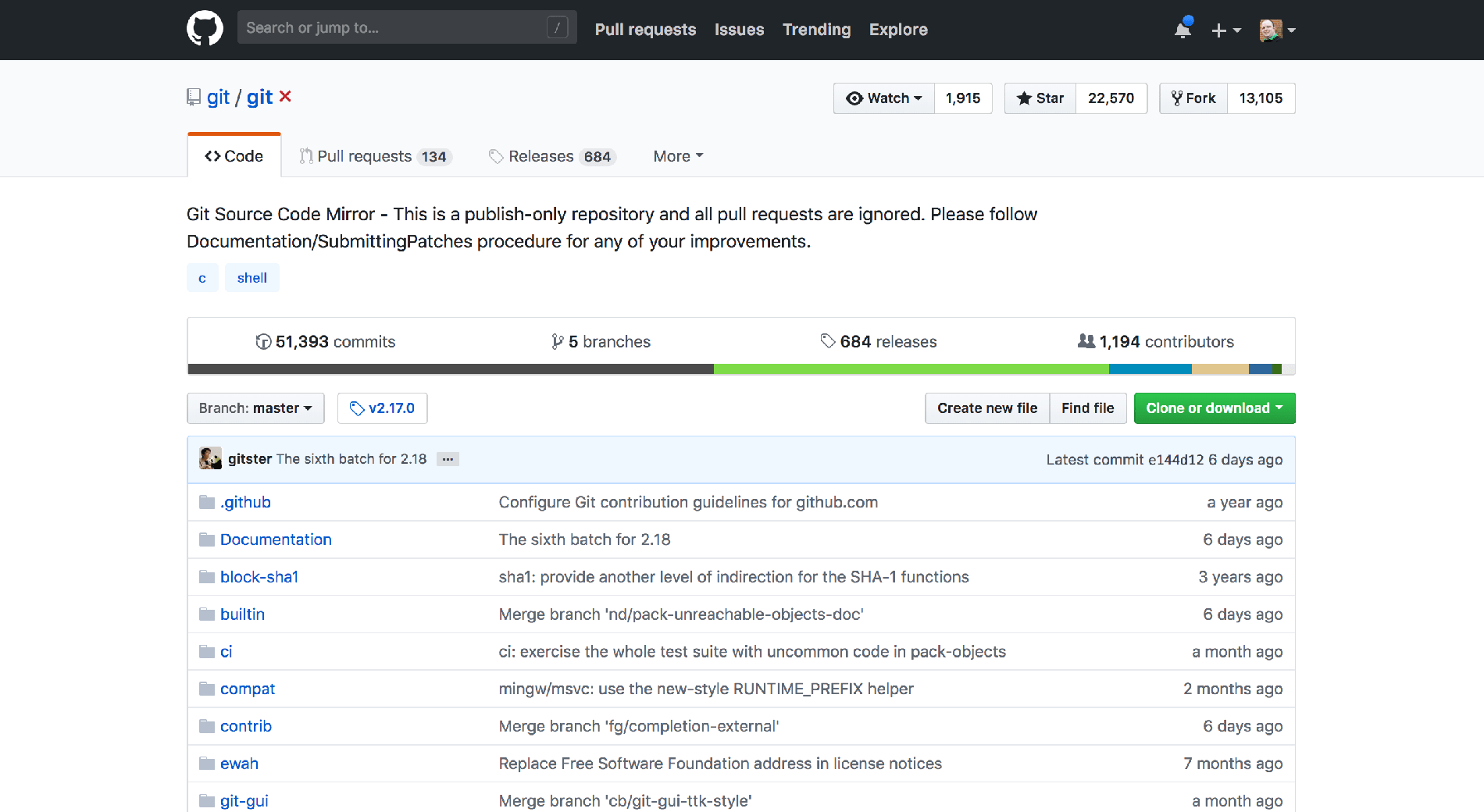**Detailed Screenshot Description:**

This image is a detailed screenshot of a web page featuring a predominantly black header. On the left side of this header, a white circle encloses a black icon of a cat. Adjacent to this icon, a dark gray search box with light gray placeholder text reads "search or jump to...". To the right within this search box, a darker gray square with rounded corners is outlined thinly in light gray, showcasing an italicized light gray "i" inside.

Moving rightwards beyond the search box, there is an array of white text labels, which includes "Pull requests," "Issues," "Trending," and "Explore". Following a gap of negative space, a white bell icon with a blue orb located at its top-right corner is displayed. Progressing further right, a white "+" icon with a white arrow pointing downwards appears, closely followed by a square profile picture with rounded corners featuring an image of a person. This profile picture also includes a white arrow pointing downwards on its right side.

Below the black header, a secondary light gray header can be observed. In its top left corner, a medium gray book icon featuring a bookmark at its bottom stands out. Positioned next to this icon is the blue text "get," followed by a black slash, and another bold blue text "get." Further right, a red "X" appears. Following this, there is some negative space, after which various rectangular buttons are displayed. These buttons consist of light gray gradient boxes, lighter at the top and darker at the bottom, and are linked to white boxes. Inside the gray boxes, black text and icons can be identified, while the white boxes contain black numbers.

There are three sets of these buttons:
1. The first set displays an eye icon labeled "Watch," a black triangle pointing downward, and the number "1915."
2. The subsequent sets follow a similar design fashion with varying icons and numbers. 

This intricate setup provides a clear and organized visual representation of the web page layout.